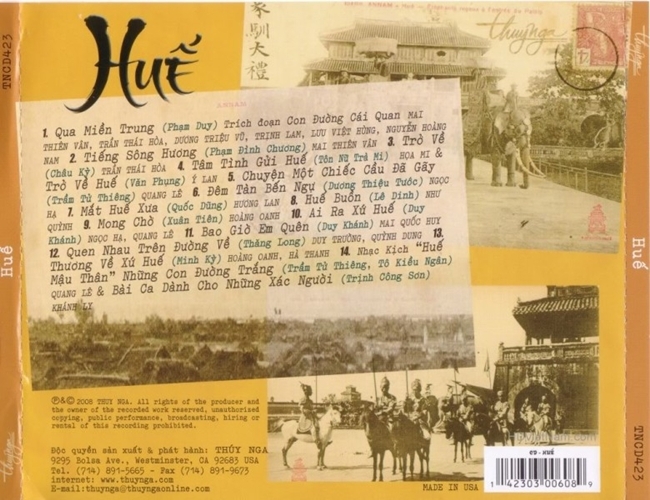The image likely depicts the back cover of a music CD or a book related to Chinese history or culture, distinguished by its vibrant orange and yellow background. Central to the design are a series of overlapping black and white photographs portraying historic scenes, including men on horses, a temple, warriors, and an elephant in front of a building, indicative of ancient Asian settings. Prominent on the cover is the word "HUE," displayed in large black letters with a distinctive mark above it. Below this, there's text that appears to be a track listing written in Chinese script, underlining the theme of the content. Additional details such as a barcode in the lower right corner and the label "Made in USA" suggest this item is prepared for sale. A side panel or spine on the left and right reiterates "HUE" in both orientations, enhancing its visibility. The overall style fuses visual scenes of historical significance with textual information, creating a compelling advertisement or artistic piece rooted in Chinese heritage.